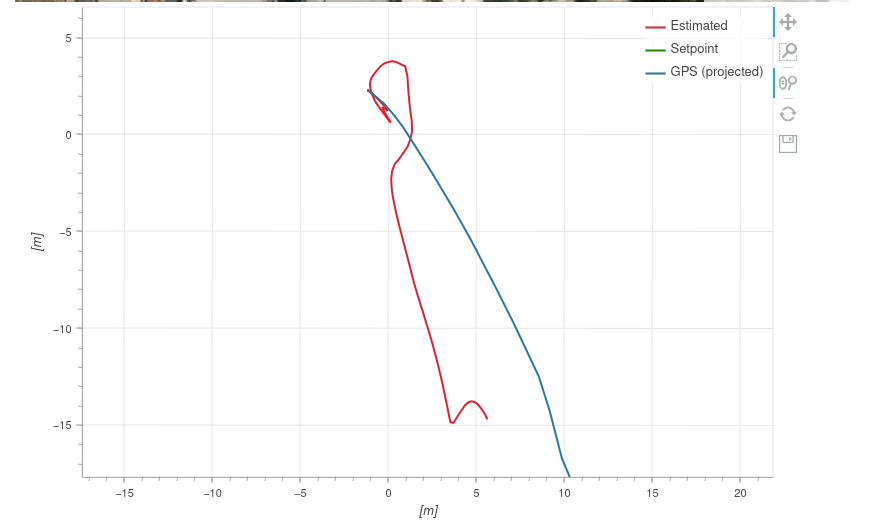The image features a graph with axes labeled in meters, indicated by parentheses around lowercase m. The x-axis spans from -20 to 20 in increments of 5, while the y-axis ranges from -20 to 5, also in increments of 5. The graph has a grid pattern in the background created by light gray lines forming squares. In the upper right corner, a legend describes three solid lines: a red line for "Estimated," a green line for "Set Point," and a blue line for "GPS Projected." The red and blue lines, representing estimated and GPS projected paths respectively, visually capture attention with their unusual, looping trajectories. They intersect and cross each other multiple times, finally converging near the zero mark on both axes.